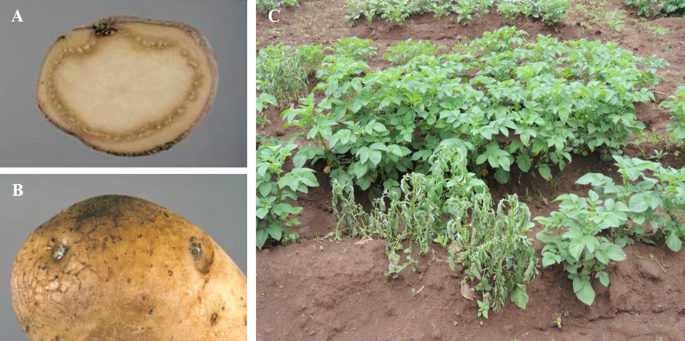The image is a mosaic consisting of three photos labeled A, B, and C. Photo A, situated on the top left and occupying one-third of the left side, features a potato that has been cut open to reveal its beige interior with circular marks and a solid gray background. Photo B, located below A, depicts the outer appearance of a whole potato with its tan skin covered in black spots. Both A and B share the left third of the image, stacked vertically. Photo C, dominating the right side of the image as a large square, captures a top-down view of a garden. It showcases a plant with small green leaves sprouting from brown soil, symbolizing the potatoes being cultivated. The three photos collectively illustrate the different stages and perspectives of a potato—from its interior and exterior to its growth in a garden.